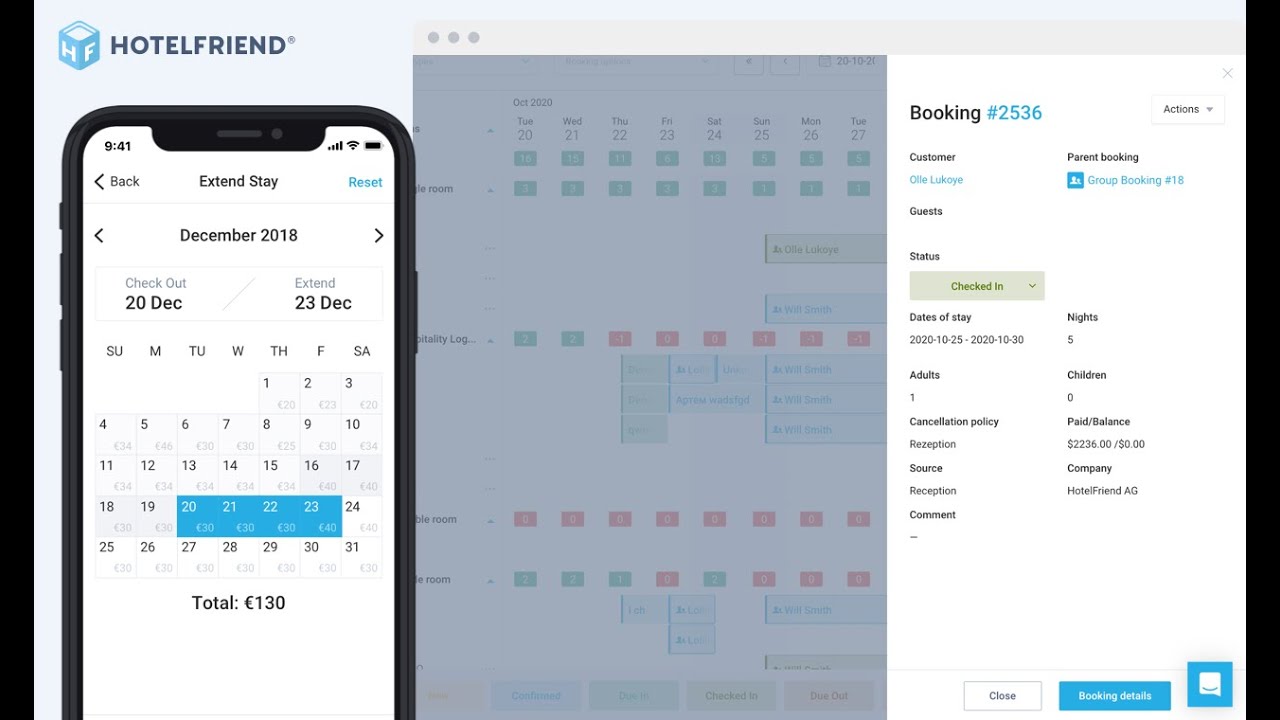This is a detailed screenshot depicting an interface from a software named "HotelFriend". The interface is divided into three vertical sections.

On the left, there is an image of a smartphone displaying an option to extend a hotel stay. It reads "Extend Stay, December 2018, Check-out 20 December / Extend 23 December." A calendar is shown highlighting the dates December 20th, 21st, 22nd, and 23rd in blue, each marked with a cost of 30 euros, accumulating to a total of 130 euros.

The middle section contains a grayed-out calendar image, making it somewhat difficult to discern the specific details or focus points of this area.

The right section features a white background with booking details at the top. It reads, "Booking #2536, Actions," followed by customer details: "Customer: OLLE LUKOYE," "Parent Booking," "Group Booking #18," "Guests," "Status: Checked In," "Dates of Stay: 2020-10-25 through 2020-10-30," "Nights: 5," "Adults: 1," "Children: 0," "Cancellation Policy," "Paid / Balance," "Reception: 2236 / 0," "Source: Company," "Reception," "Hotel Friend AG," and a comment section labeled "Close Booking Details."